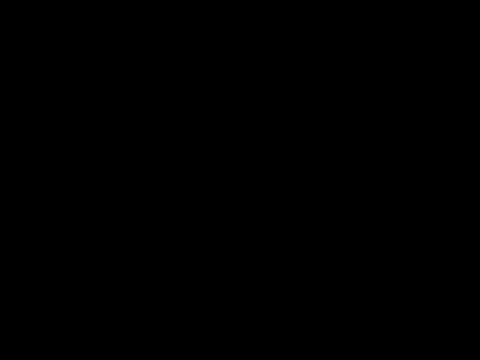The image presents a uniformly black rectangle, slightly longer than it is tall, with very sharp edges, neatly centered against a white computer screen background. The entire image is devoid of objects, text, and any other color or details, embodying a pure, solid black with no visible variations or gradations. It’s not the deepest black possible, but it distinctly avoids any shades of gray or other modifications, ensuring a seamless, uninterrupted blackness. The scene captures nothing beyond this simple yet striking depiction of a black rectangle.